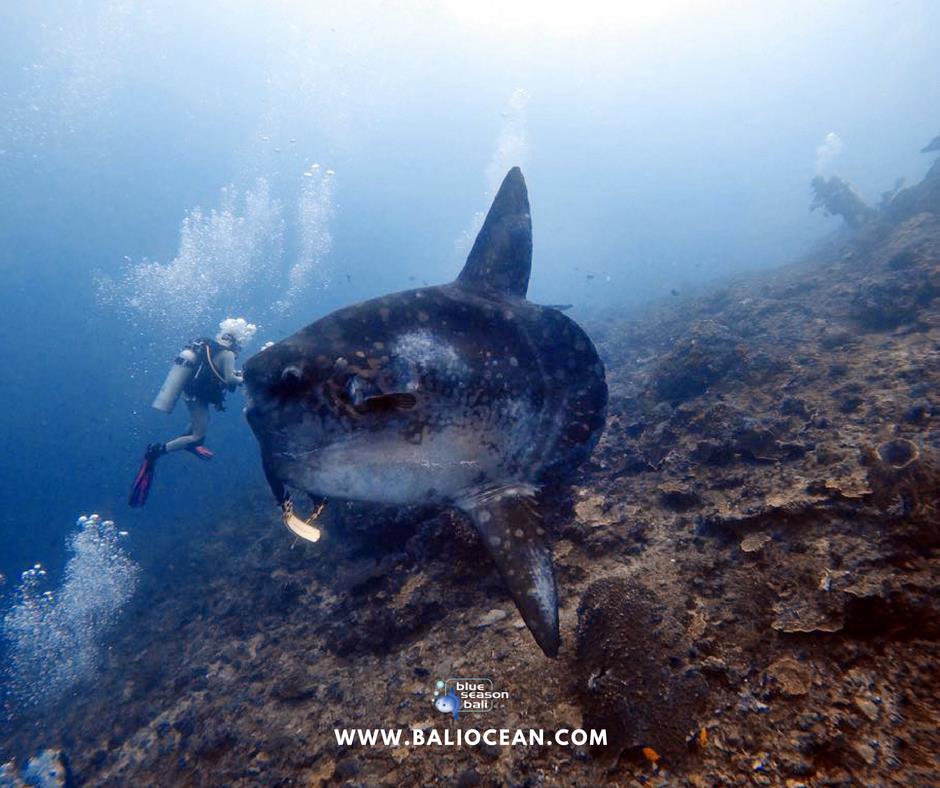This underwater color photograph captures the mesmerizing scene of a vast, oceanic world. At the focal point is an enormous, bullet-shaped fish, possibly a shark or whale, resting horizontally on a seabed composed of tan, brown, and black rocks, which could also be dirty brown coral. This massive fish, with only its head and two prominent fins clearly visible, dominates the composition. A scuba diver equipped with a tank and flippers approaches from the front, their position accentuated by a flurry of air bubbles escaping from their gear. The diver's presence juxtaposes against the enormous scale of the fish, which dwarfs them significantly. Additionally, the legs of another diver are faintly discernible behind the fish, and near the top right, a blurred hint of possibly another diver can be seen, adding depth and activity to the underwater scene. Notably, attached to the fish is something gold, the nature of which is indistinguishable. The bottom of the image is overlaid with white text, displaying the logo and words "Blue Season Bali" along with the website "www.baliocean.com," anchoring the image in its marine exploration context.